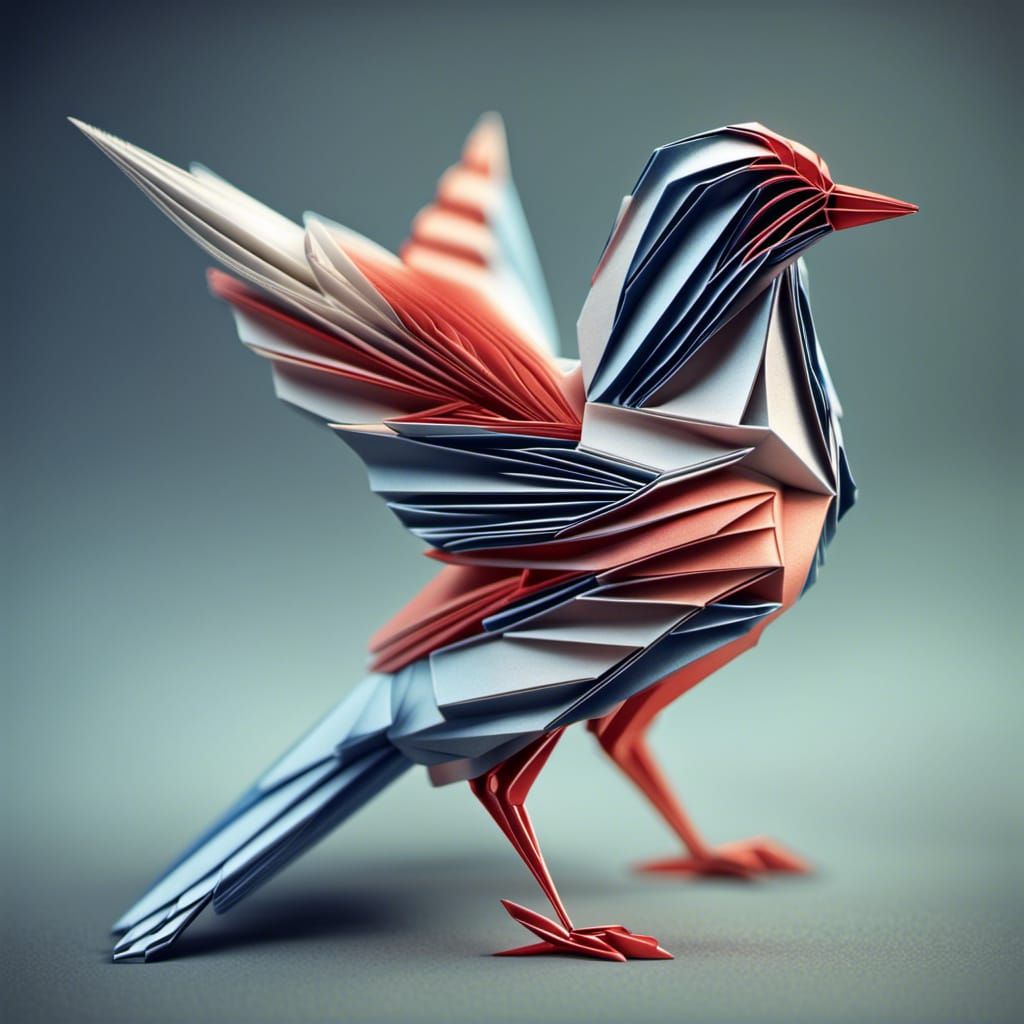This close-up photograph captures an intricately folded origami bird, resembling an eagle, made entirely from paper with an American flag motif. The paper features solid red, white, and blue sections, along with an area of red and white stripes, which emphasize the flag-themed design. The bird, marked by its vivid colors, has its beak and feet in red, and its body primarily in blue, although some of the over feathers show red. The wings are a striking combination of red, white, and blue, with the left wing, slightly out of focus in the background, displaying distinct red, white, and blue stripes along the front part. The craftsmanship is impeccable, with fine pleats giving an appearance akin to real feathers. The bird is depicted in a sitting position with its wings splayed behind it and its legs providing support. The background gradient transitions from dark blue at the top to lighter blue at the bottom, adding depth to the image. The bird faces to the right, standing on a surface, emphasizing the elaborate and time-consuming effort that went into creating this stunning paper sculpture.